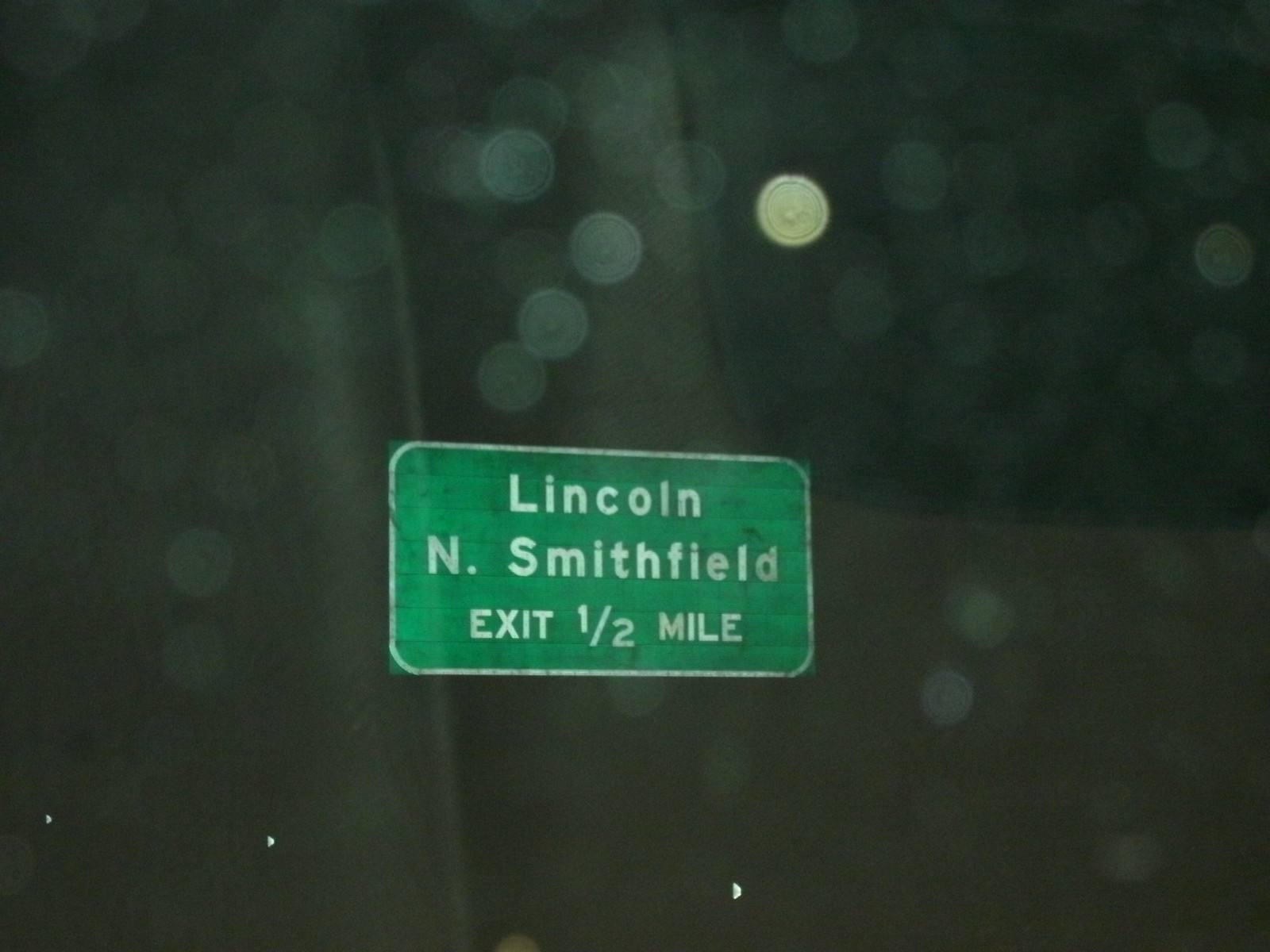A nighttime photograph taken through a rain-spattered vehicle window captures a green street sign with a white border. The sign, slightly blurred due to raindrops clinging to the window glass, reads "Lincoln" in large white letters at the top center. Below it, the sign displays "N. Smithfield" with a dot after the letter "N," and in a smaller font beneath that, it indicates "Exit ½ Mile." In the upper right corner of the image, a particularly bright, circular blur suggests the presence of a street light, adding to the atmospheric conditions of the rainy night.